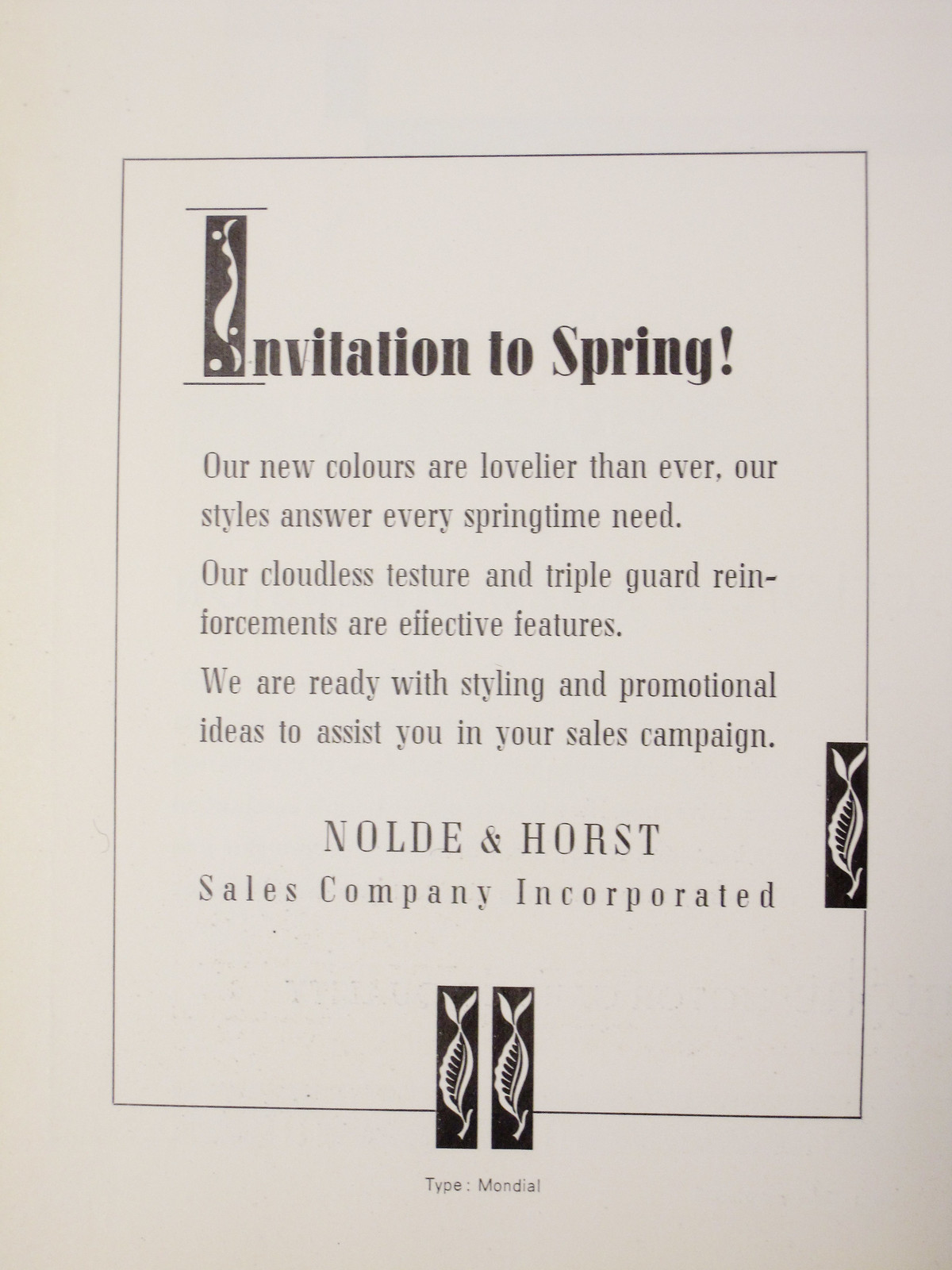This image features an elegantly designed invitation card with the title "Invitation to Spring!" prominently displayed at the top. The card, which is a promotional piece from the Nodae and Horst Sales Company Incorporated, boasts of their new spring collection with the phrase "Our new colors are lovelier than ever" and "Our styles answer every springtime need." It highlights their effective features, including "cloudless texture" and "triple guard reinforcements." The card reassures potential clients with a message promising readiness with "styling and promotional ideas to assist you in your sales campaign." The design is set against a simple white background with black text and includes black and white rectangular images, all enclosed within a thin black border, reflecting a minimalist yet refined aesthetic.